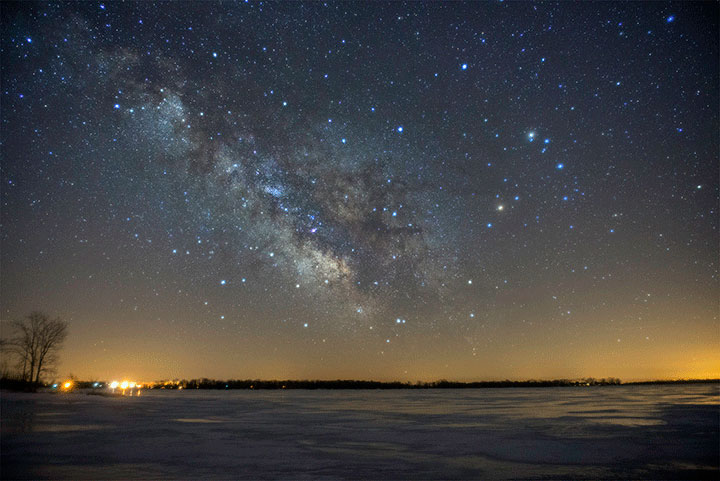In this night scene, the vast and star-lit sky dominates about three-quarters of the image, showcasing the Milky Way galaxy stretching diagonally from the top left towards the center. The sky is filled with bright, scattered stars of varying sizes and shapes. Below the celestial expanse, the horizon glows with a yellow-orange hue, devoid of stars, and is marked by a distinct black line formed by a row of leafless trees. To the left side, lights possibly from a city or passing cars illuminate a taller, nearer tree with no leaves. The foreground features a shimmering, bluish-gray lake reflecting the star-speckled sky while snow gently falls. Descending through the middle, a smoky, brownish-veined shape with a white haze adds a mystical touch to this serene, ethereal landscape.